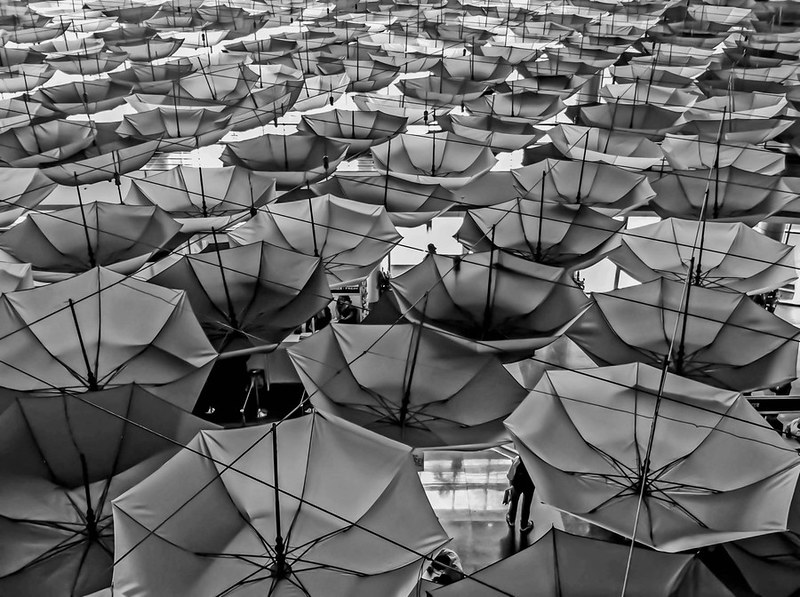This surreal, black-and-white image presents a captivating, somewhat disorienting scene: an entire field of upside-down umbrellas, their handles jutting upwards towards the sky. The umbrellas are meticulously arranged in rows and columns, creating a structured yet chaotic visual. Each umbrella, open and inverted as if to catch the rain from above, dominates the close-up frame, leaving no clear view of the sky. The handles of these umbrellas appear to be intertwined or perhaps supported by wires or thin poles, giving a semblance of being connected in a deliberate pattern.

Amid this sea of umbrellas, glimpses of a wet sidewalk and the feet and legs of passing pedestrians are visible through the narrow gaps, hinting at activity below. Faint light seeps through from underneath, suggesting the presence of buildings or streetlights illuminating the scene from beneath the canopy of umbrellas. The perspective of the photo brings an intriguing vantage, almost as if taken from an elevated position looking down, further enhancing the surreal and artistic quality of the composition.